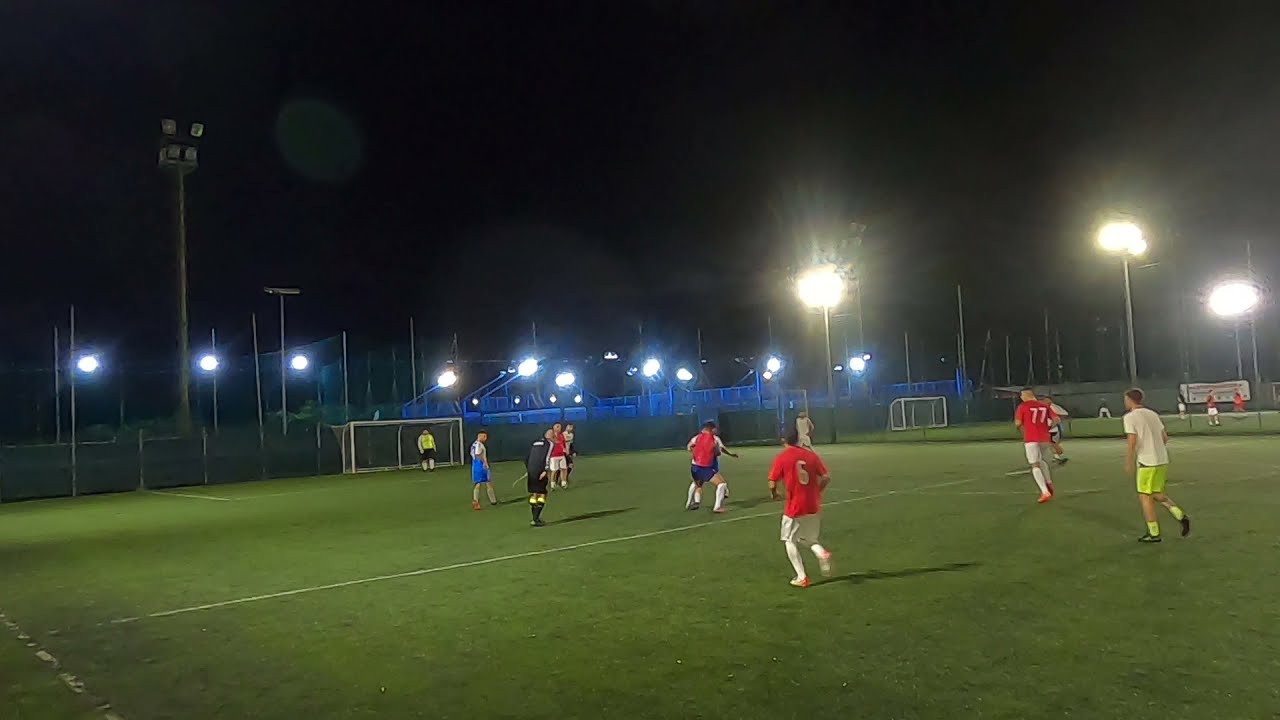The photograph captures a nighttime soccer game under a black sky illuminated by bright, fluorescent lights mounted on tall poles. The green field, though somewhat worn with faded white stripes, stretches out in front of the viewer. The scene prominently features two teams: one team in red jerseys with white numbers—players numbered 6 and 77 are particularly noticeable—and the other in white jerseys paired with various colored shorts. Notable among the players are a referee in black, a player in white with neon green shorts and socks, and another in blue shorts. The goalie, situated to the left of the image, wears a yellow jersey and black shorts. In the background, a blurry, wire fence separates the field from the stands, which appear to be empty or indistinct. Another active game is visible on an adjacent field to the right, adding dynamic layers to the scene. Far off near the fence, a few people are faintly discernible, though it's unclear if they are watching the game.